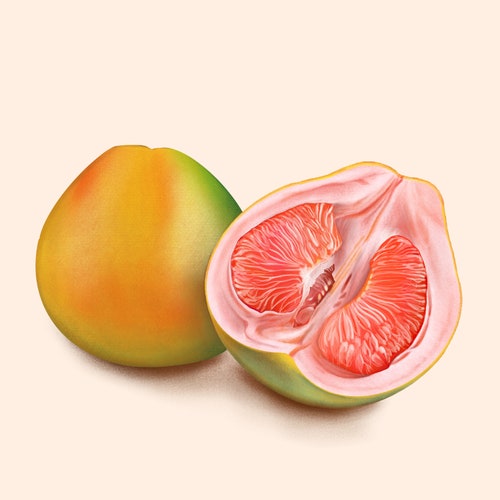The image features a highly detailed and vivid illustration of a citrus fruit against a light pink background. At the center of the composition is a whole, slightly ovular fruit displaying various shades of orange and red, blending with light and dark green hues, particularly towards the edges. This fruit is depicted whole on the left side and has a somewhat plump shape with a mix of lighter and darker colors creating a textured, lifelike appearance. To the right of this whole fruit, a second fruit is shown cut in half, revealing its intricate interior. The inside of the halved fruit displays a light pink flesh with darker orange segments that are reminiscent of tangerine wedges, holding a few seeds. The meticulously illustrated segments offer a striking contrast against the vivid pink interior, resembling a grapefruit, although the exact type of citrus is not definitively identified.